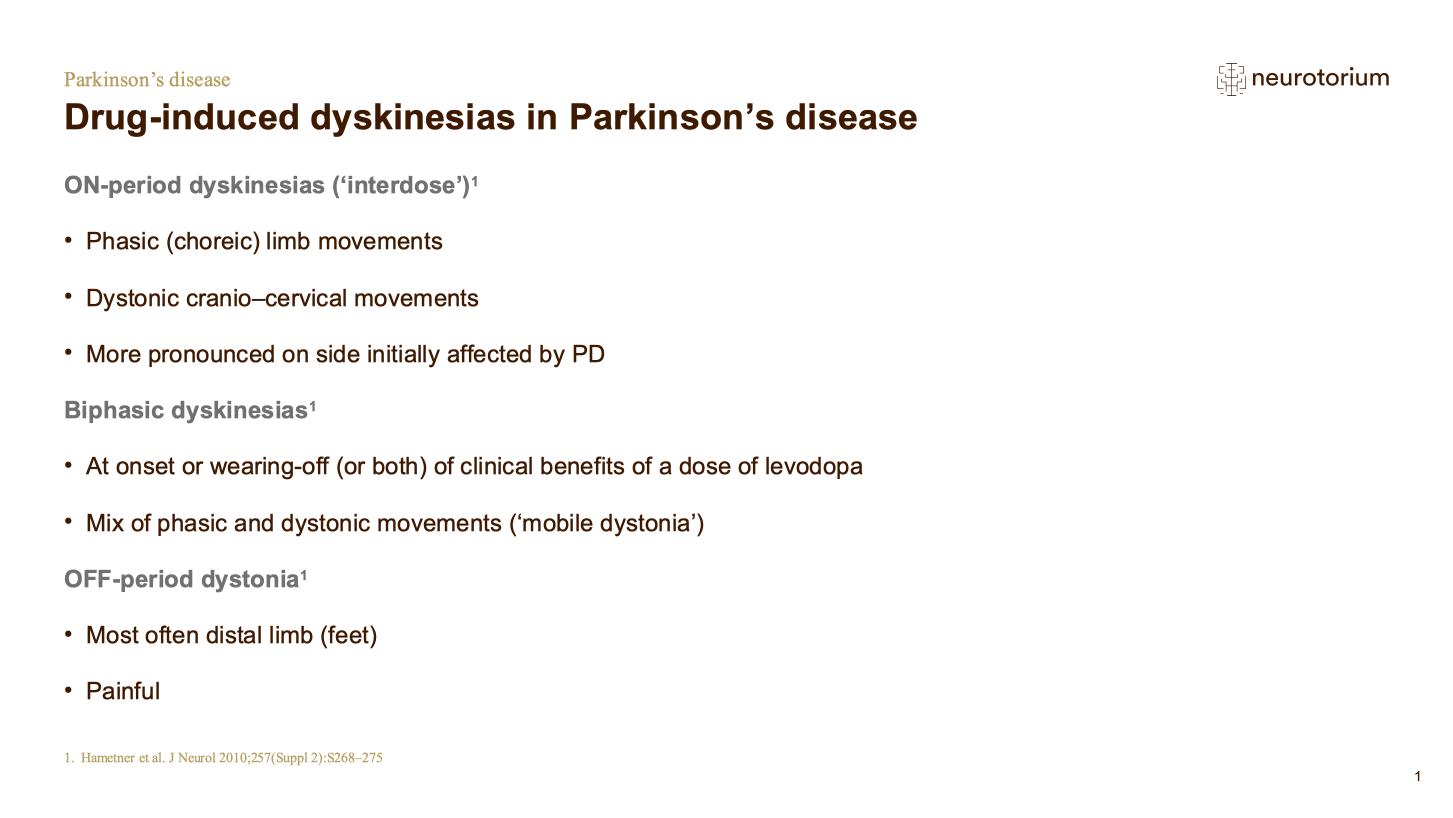Certainly! Here’s the cleaned-up and more detailed caption:

---

This image is a screenshot from the webpage titled "Neurotorium." The logo and brown text are positioned in the top right corner on a white background. At the top left corner, the text reads "Parkinson's disease and drug-induced dyskinesia."

Under the main heading, there is a subtitle specifying "On-period dyskinesia" with a citation marker "[1]." The content below this subtitle includes three bullet points describing symptoms associated with on-period dyskinesia:
- Phasic (choreic) limb movements.
- Dystonic cranial and cervical movements.
- Symptoms are more pronounced in areas initially affected by Parkinson's Disease (PD).

Next, a subheader titled "Biphasic Dyskinesia" appears. Below this are two bullet points explaining the characteristics:
- Occurs at the onset or wearing off (or both) of the clinical benefits of a dose of levodopa.
- Consists of a mix of phasic and dystonic movements (mobile dystonia).

Another subheader, "Off-period Dystonia," follows, with two bullet points outlining its characteristics:
- Most often affects distal limbs, particularly the feet.
- Painful.

At the bottom, there is a citation from Hapner et al., found in the "Journal of Neurology," providing detailed reference information for the source of this content.

---

This caption provides a structured and detailed summary of the information displayed in the screenshot.